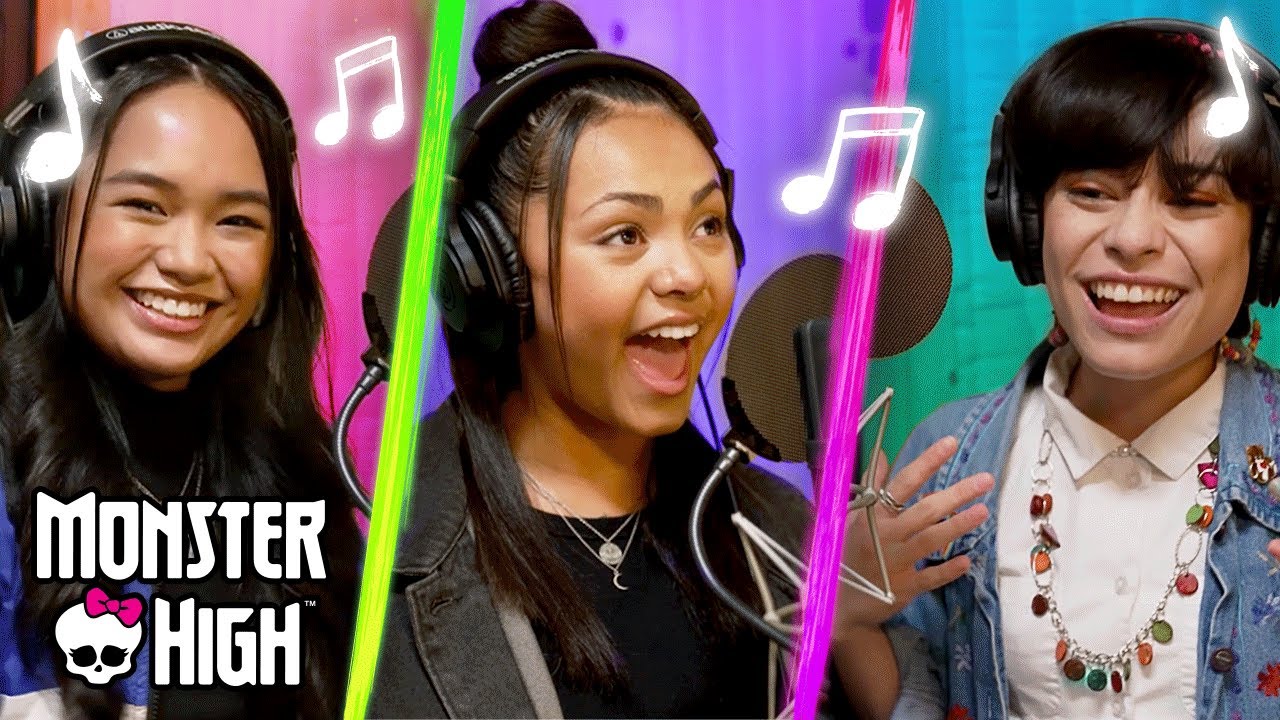The image appears to be a thumbnail or promotional content, likely for a Monster High project, showcasing three individuals separated by colorful lines. On the left, a woman with black hair and a cheerful expression stands against a pink background, wearing headphones and partially visible upper-body attire, with the "Monster High" logo, including a skull with a pink bow, at the bottom of her section. In the center, another woman, energetically singing or shouting into a microphone with an open mouth, is set against a purple background. She wears black headphones, a black T-shirt, and a gray jacket. The rightmost side features a figure who might be a boy or a girl, dressed in a white shirt under a blue jacket, a distinctive necklace, and headphones. This person's background is blue, and they appear to be holding their hand up to the side. Music notes are scattered throughout the image, further suggesting the theme of recording or singing. Green and purple lines separate these segments, enhancing the vibrancy and connection between the different parts of the montage.